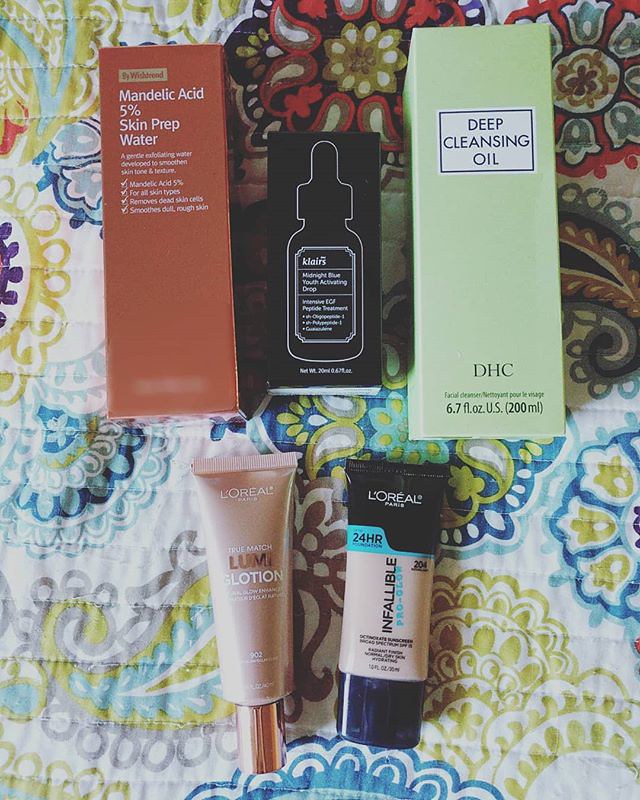The image features a neatly arranged collection of skincare products displayed on a cloth surface that resembles a bed quilt or blanket. The photograph is taken in close-up, capturing the entirety of each item in detail. 

At the top of the arrangement, there are three boxed products. The first box on the left has a brownish tint with white lettering that reads "Mandelic Acid 5% Skin Prep Water." Next to it, in the middle, is a smaller black box with a white outline of a dropper bottle on the front. The label on this box reads "Tlars," though some of the smaller text is illegible. The third and largest box on the right has a light green covering and is labeled "Deep Cleansing Oil" in dark letters on a white background within a rectangular box at the top. Towards the bottom of this box, the brand "DHC" is visible along with the volume of the product, "6.7 fluid ounces (US) / 200 milliliters."

Below these boxes, two smaller, unpackaged tubes are placed side by side. The tube on the left appears to be a dull pink color and is labeled with "L'Oreal" at the top in white letters. Among the text on the front, the words "Loom Lotion True Match" are discernible. The tube is topped with a silver cap. To its right is a cylindrical product, also by L'Oreal, labeled "24-hour Infallible Pro Gloss." This tube, unlike the others, is more cylindrical in shape.

Each product is carefully positioned to show its design and branding clearly, creating a detailed and visually informative arrangement.